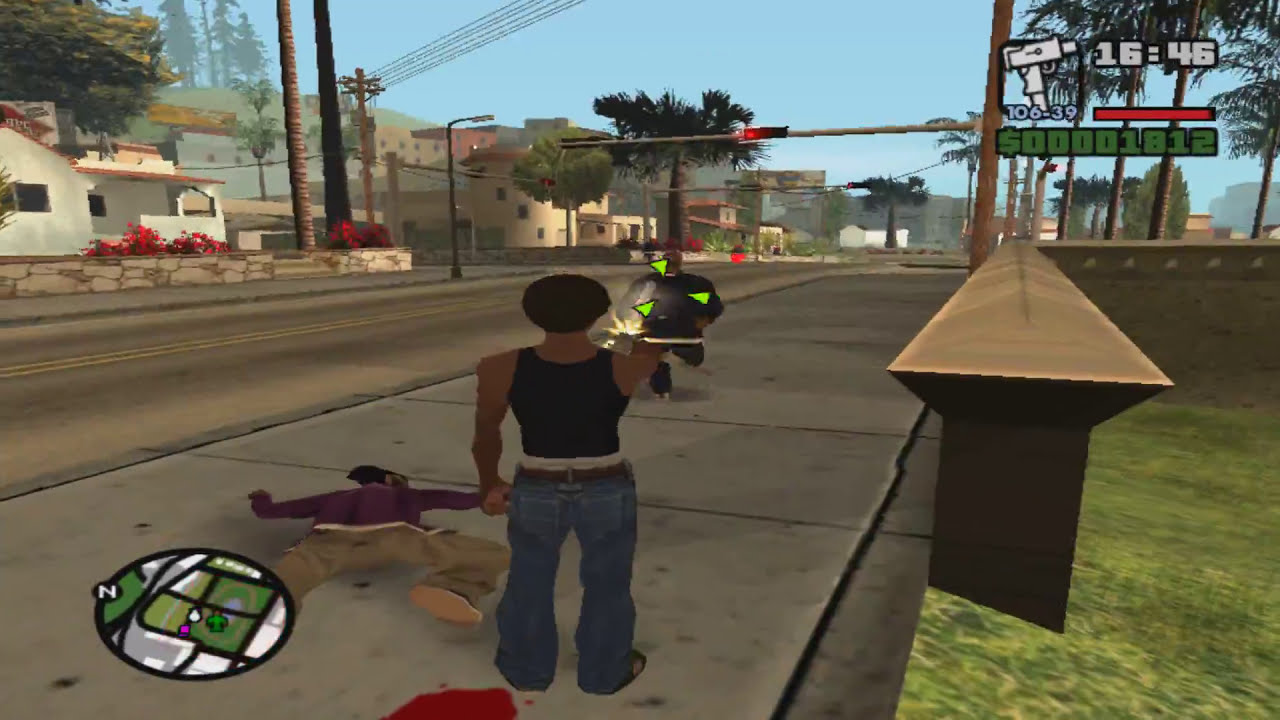The image is a detailed, colorful illustration, landscape in orientation, depicting a still frame from a violent video game set in a city. In the center, an African-American male with dark skin and hair, wearing blue jeans and a black tank top, stands on the sidewalk. He is seen firing a gun, indicated by a flashing light from his outstretched hand, aimed at another figure who appears to be running toward him. The gunfire is underscored by three green targeting triangles on the approaching figure.

To the left of the shooter, a man wearing khakis and a purple shirt lies face down on the sidewalk, arms and legs outstretched, with a puddle of blood behind him, suggesting he is mortally wounded. The backdrop features palm trees, power lines, and California-style houses on a hillside, contributing to an unmistakable West Coast ambiance. A straight intersection with a stoplight and streetcar tracks runs adjacent to the scene. Additionally, the lower-left corner of the image displays an inset map with an "N" indicating the player’s location within the larger city.

The upper right corner of the screen displays a gaming timer set at 16:46, alongside a score of $1812, further emphasizing the video game's environment. Across the street, white stucco buildings with red flowers and other storefronts are visible, contributing to the urban, scenic background.